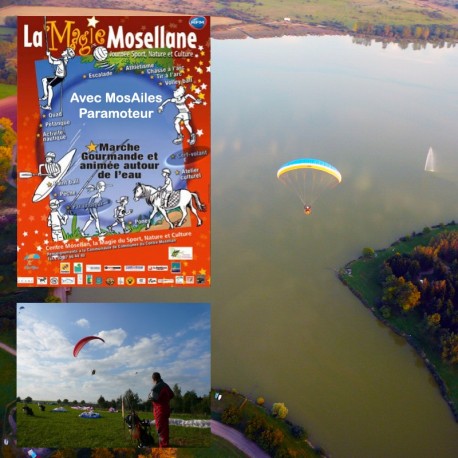The image is a detailed composite scene with a primary focus on a photograph capturing an aerial view of a river. Centered in this photograph is a parasailer gliding over the murky, dark water, which has a green tinge to it. The parasail stands out vividly with its bright yellow and turquoise colors. To the right of the parasailer, a sailboat navigates the river.

Superimposed on the left side of the main photograph are two additional frames. The top left frame features a colorful red magazine cover, titled "La Magique Mousselin," adorned with illustrations of various outdoor activities such as horseback riding, walking, and climbing, seemingly animated and lively. Beneath this, though not exactly in the bottom left corner, is another smaller photograph capturing a glider, viewed from the ground against a backdrop of blue sky. Both additional frames contribute to the dynamic and adventurous theme of the composite image.